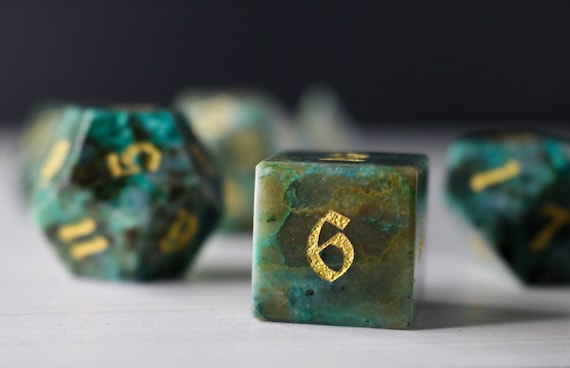The image showcases a set of stone-like dice against a beige background. The main focus is a six-sided die positioned at the forefront, crafted from a polished, greenish-blue marble-like stone with intricate patterns of green and light brown. The number six, depicted in a stylized gold font, is prominently visible on its front face. Adjacent to this cube, slightly to the left and set in the background, is a twelve-sided die, though its edges are blurred, emphasizing its secondary importance in the composition. This die displays numbers such as five, eleven, and possibly a six or nine, all rendered in similar golden numerals. To the right of the image, there appears to be another faceted die, potentially a ten-sided one, although the exact configuration is unclear due to the image's blurred background. This die also features numbers, including a one and seven. The overall impression is one of elegantly crafted game pieces, each differing in shape yet unified by their polished stone aesthetic and gold-embellished numbers.